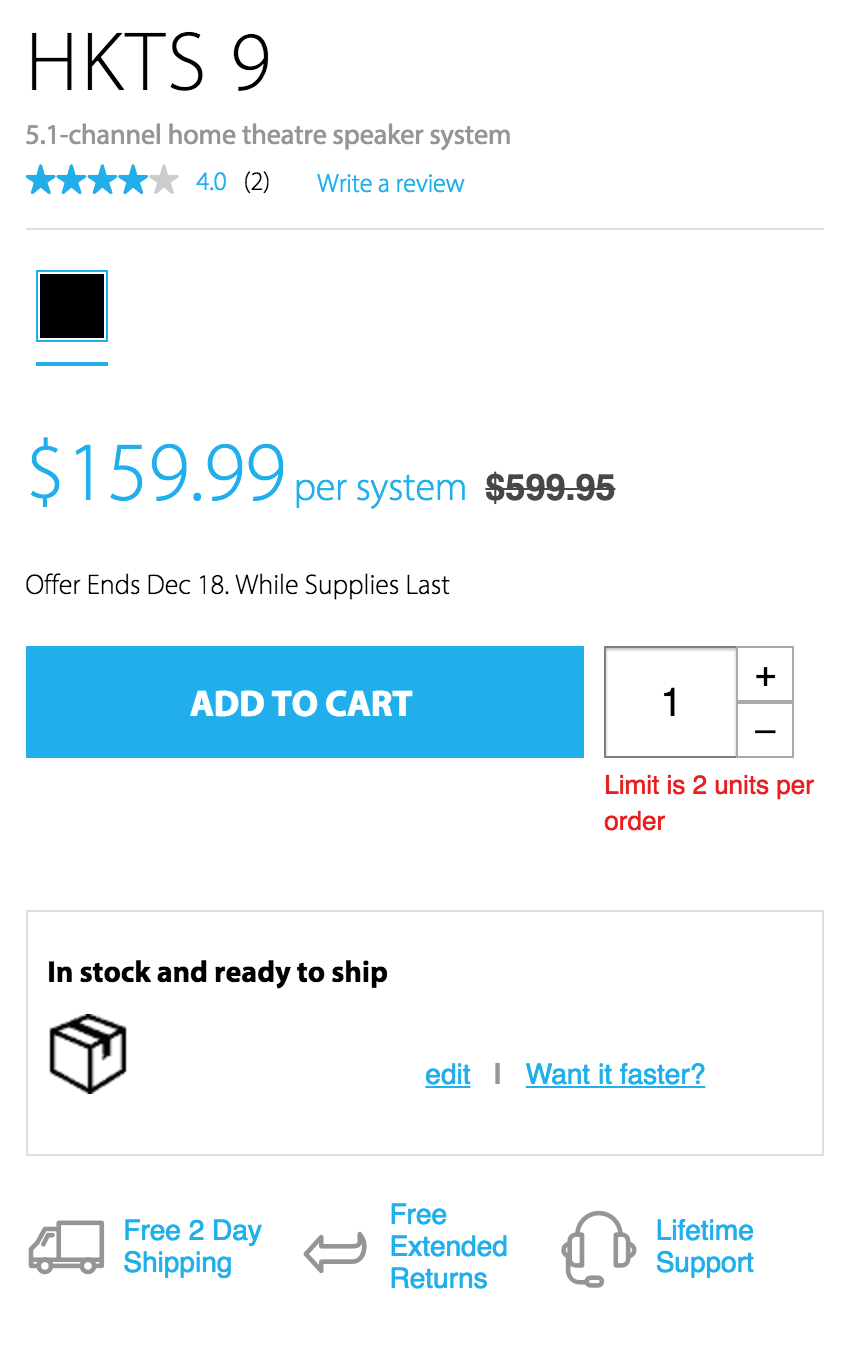Certainly! Here is a cleaned-up and detailed caption for the described image:

---

Screenshot of an online shopping site featuring the Harman Kardon TS 9 5.1 Channel Home Theater Speaker System. The product has a rating of four stars out of five. Originally priced at $599.99, it is currently on sale for $159.99 per system. The blue text indicates this offer is valid until December 18th while supplies last. Below, an "Add to Cart" button is highlighted in blue with an adjacent quantity adjustment box limited to two units per order, which is marked in red. The product is listed as in stock and ready to ship, with an icon indicating free two-day shipping. There are additional perks such as free extended returns and lifetime support.

---